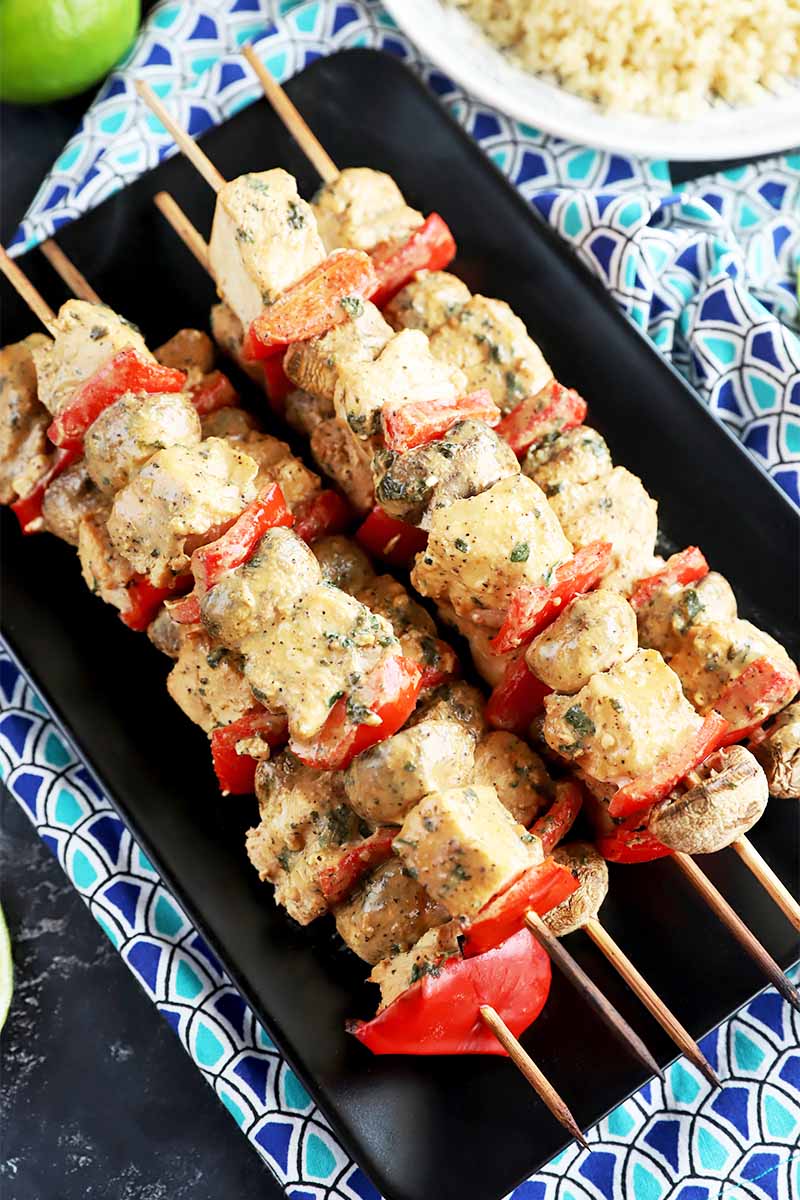This photograph features a tantalizing display of shish kebabs, meticulously arranged on wooden skewers. Each skewer follows a decorative pattern, starting with thick, juicy pieces of meat or possibly tofu, interspersed with vibrant red bell peppers and succulent tomatoes. Some skewers also include plump mushrooms, adding an earthy flavor to the ensemble. The kebabs are generously coated in a cheesy marinade with green herb flecks, enhancing their visual appeal and suggesting a rich, savory flavor.

There are approximately six skewers, all resting atop a sleek black tray. The tray sits on an intricately patterned turquoise and dark blue tablecloth, bordered in black and white, which adds a touch of elegance to the presentation. The char marks on the vegetables indicate the kebabs have been freshly grilled, likely over an oblong, stove-like metal setup not visible in this shot. In the photograph's top corners, just slightly cut off, are glimpses of a green lime to the left and a plate of rice to the right, completing this delectable scene.